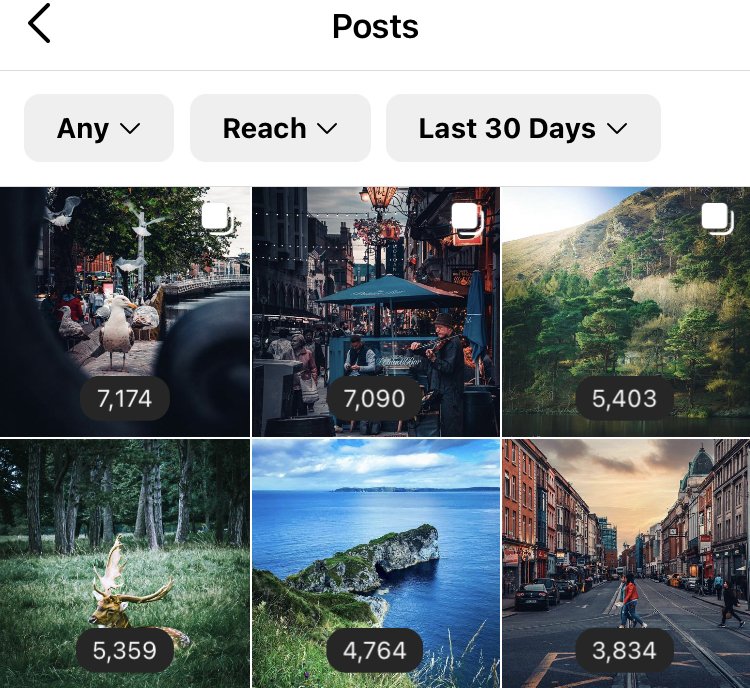The top part of the image features a white background with a black arrowhead pointing to the left. In the middle of this section, the word "POSTS" is displayed in black, all capitalized, and follows a distinct horizontal line. Below this, there are three gray rectangles. The first rectangle contains the word "Any" in black text, the second reads "Reach," and the third states "Last 30 Days." Each of these rectangles has a black downward-facing arrow on the right end, indicating that they are expandable options.

Beneath these elements are six images arranged in two rows of three. In the upper right corner of each image, there is a small white square, and at the bottom, there is a gray oval containing numerical values in white text. The numbers in the first row, from left to right, are 7,174, 7,090, and 5,403. The numbers in the second row, from left to right, are 5,359, 4,746, and 4,384.

The content of the images is as follows:
1. The first image on the top row shows a bird.
2. The second image features an umbrella and people eating at a restaurant.
3. The third image depicts a wooded area.
4. The first image on the bottom row shows a deer or moose in the woods.
5. The second image displays the ocean with a rock formation.
6. The third image captures people walking in a cityscape.